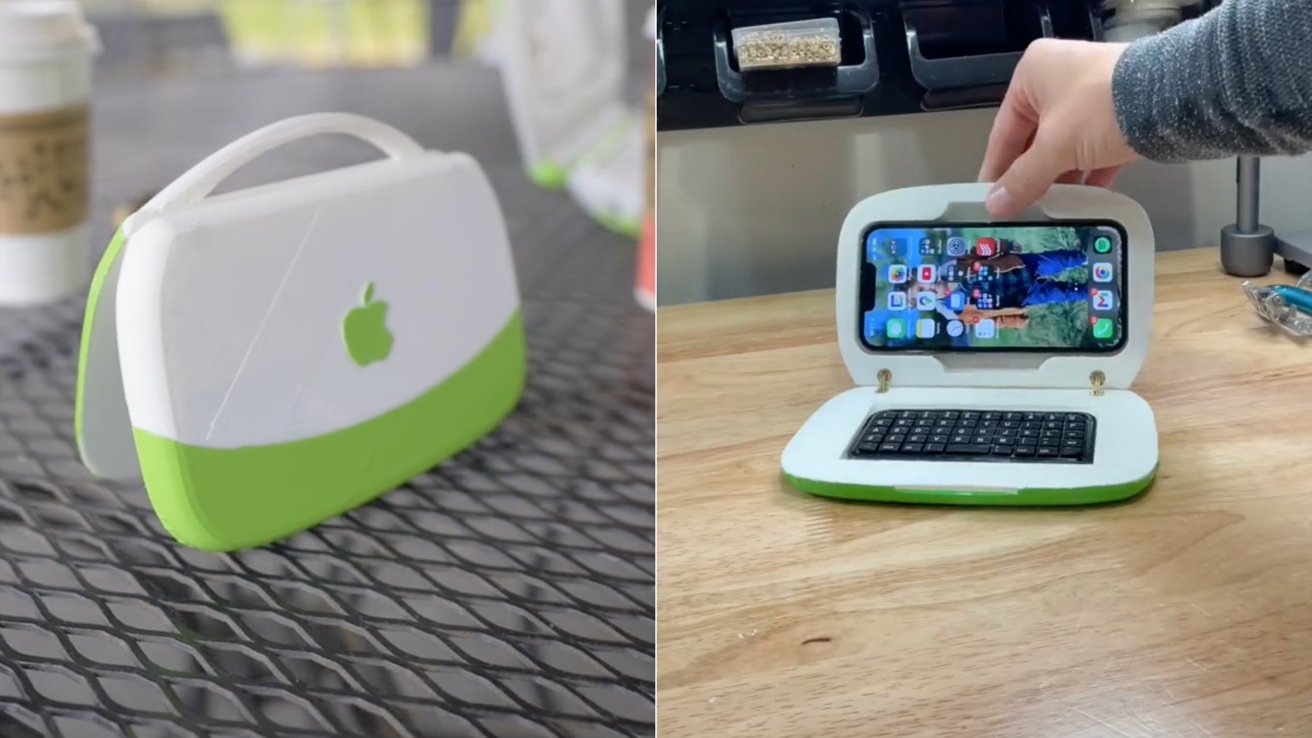This image features two side-by-side photos of what appears to be a child-friendly Apple device setup. The photo on the left shows a portable Apple device case that is white and light green, with a light green Apple logo in the center. This case, which has a handle, is resting on a metal grated table, and a coffee cup can be seen in the background. To the right, someone wearing a dark gray long sleeve shirt is holding open what seems to be a foldable Apple laptop or tablet device designed for children. The open device reveals a small keyboard and a screen, which is actually a smartphone placed into the setup. This setup is on a light wooden table, and in the background, there are black plastic baskets and what appears to be a printer with a piece of paper hanging out.